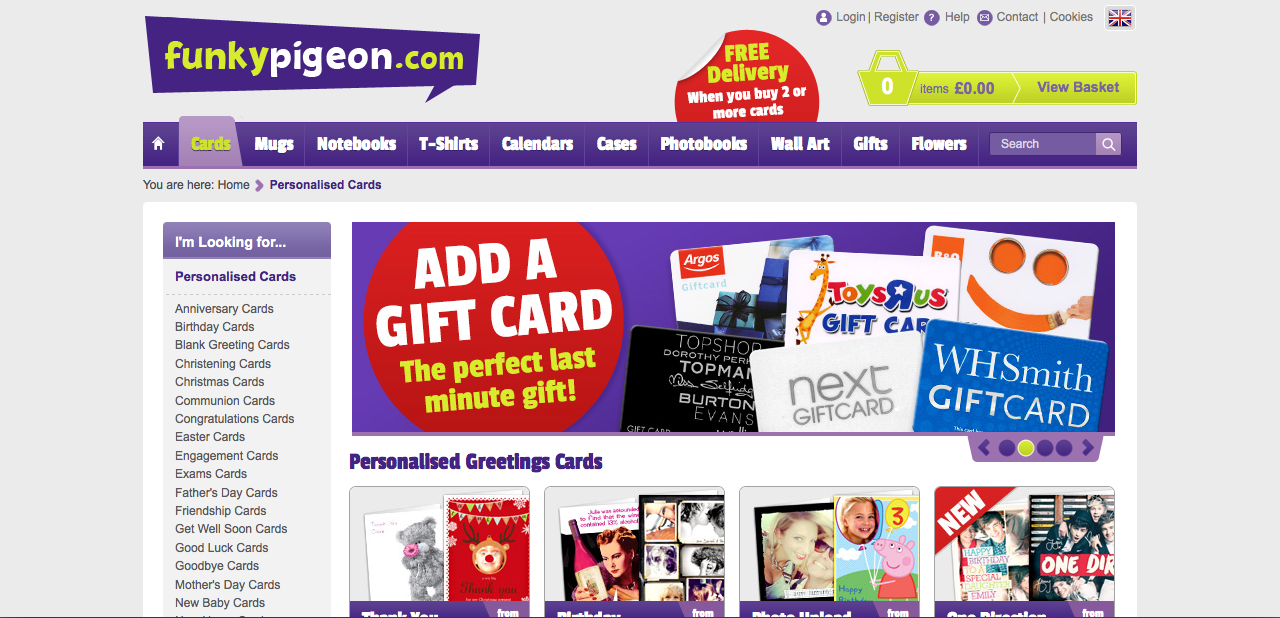This image captures a screenshot of a website specializing in the sale of various gift items, prominently featuring the logo of 'MonkeyPigeon.com' in the top left corner. Directly below the logo, a horizontal navigation menu offers categories such as cards, mugs, notebooks, t-shirts, calendars, photo books, wall art, gifts, and flowers. To the far right of this menu, a search bar is available for specific queries.

On the left sidebar of the website, a comprehensive list of categories for cards is displayed vertically. These categories include Anniversary Cards, Birthday Cards, Bank Reading Cards, Christmas Cards, Congratulations Cards, Easter Cards, Engagement Cards, Exam Cards, Friendship Cards, Get Well Soon Cards, Good Luck Cards, Goodbye Cards, Mother's Day Cards, and New Baby Cards.

Dominating the main portion of the webpage are visual examples of the various gift cards available for purchase. Some of the highlighted gift cards include a 'Next Gift Card', a 'Toys R Us Gift Card', and a 'WH Smith Gift Card'. The clean layout and organized categories suggest a user-friendly shopping experience aimed at helping customers find the perfect card for any occasion.